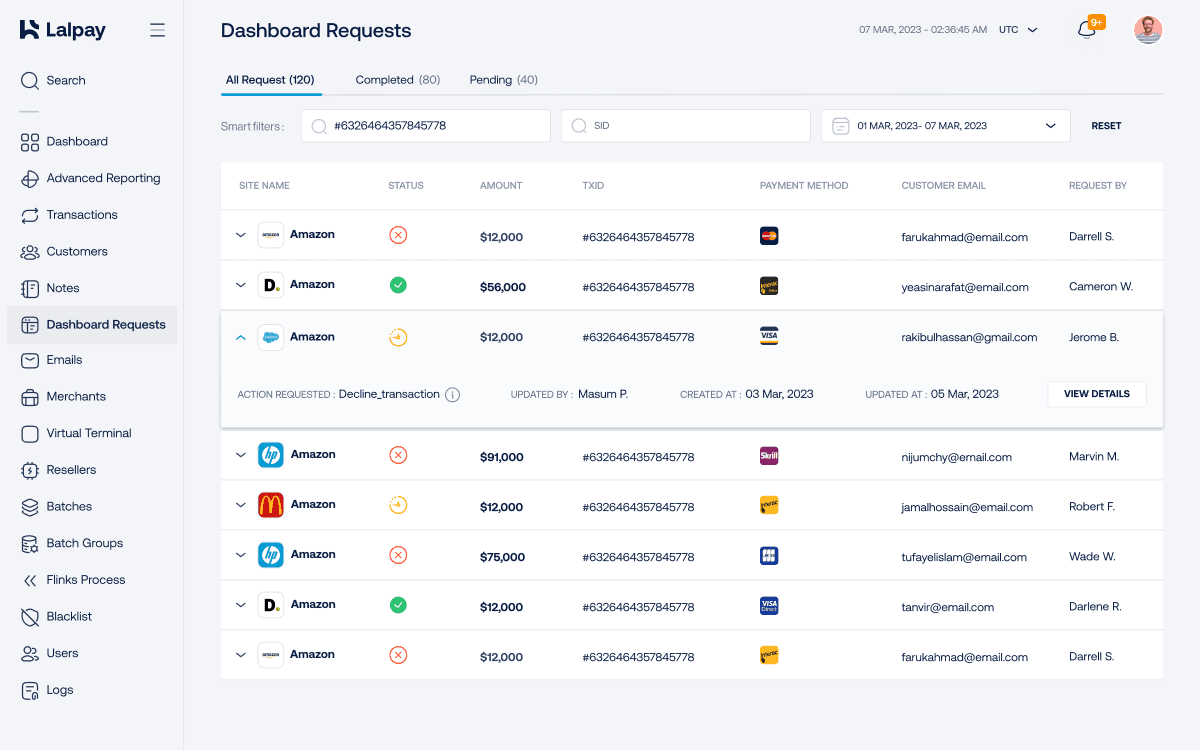A detailed screenshot of a LALPAY dashboard interface highlights various elements of the webpage. At the top left corner, the name "LALPAY" is prominently displayed. The left side of the screen features an expanded sidebar menu starting with a search bar and a magnifying glass icon labeled "Search". Below this, a comprehensive list of selectable options includes Dashboard, Advanced Reporting, Transactions, Customers, Notes, Dashboard Requests, Emails, Merchants, Virtual Terminal, Resellers, Batches, Batch Groups, Thinks, Progress, Blacklists, Users, and Logs.

The main focus is on the "Dashboard Requests" page, as indicated at the top of the display area outside the sidebar. This section contains three tabs: "All Requests" showing 120 entries, "Completed" with 80 entries, and "Pending" with 40 entries. Top right features include the current date and time, a notification bell with a count exceeding nine, and a profile picture of a man.

The "All Requests" tab is active, revealing a series of site names and associated requests. Filters are available to refine the list of requests, providing a detailed and organized view of the user's pending and completed dashboard activities.